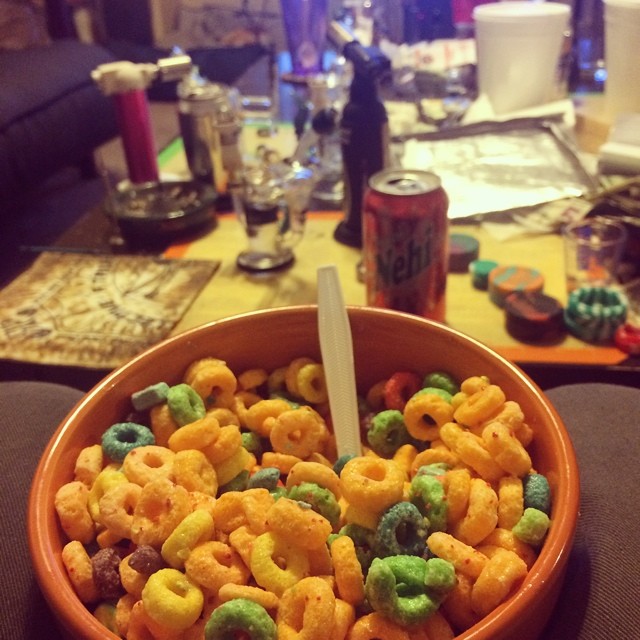In this vertical, slightly blurred photograph taken on a camera, the primary focus at the bottom of the image is an orange bowl resting on a brown sofa. The bowl contains multicolored, round cereal pieces, likely Froot Loops, in hues of orange, yellow, green, purple, and red, partially covering a white plastic spoon. Positioned in front of the bowl is a table adorned with green and orange poker chips and a red can of Nehi soda. The tabletop also hosts an assortment of blurred objects, including small handheld blow torches, a marijuana dab rig, and a small black ashtray. Additionally, the table features a patterned folded napkin, various glasses, and plastic containers, all contributing to a cluttered, yet detailed, scene.